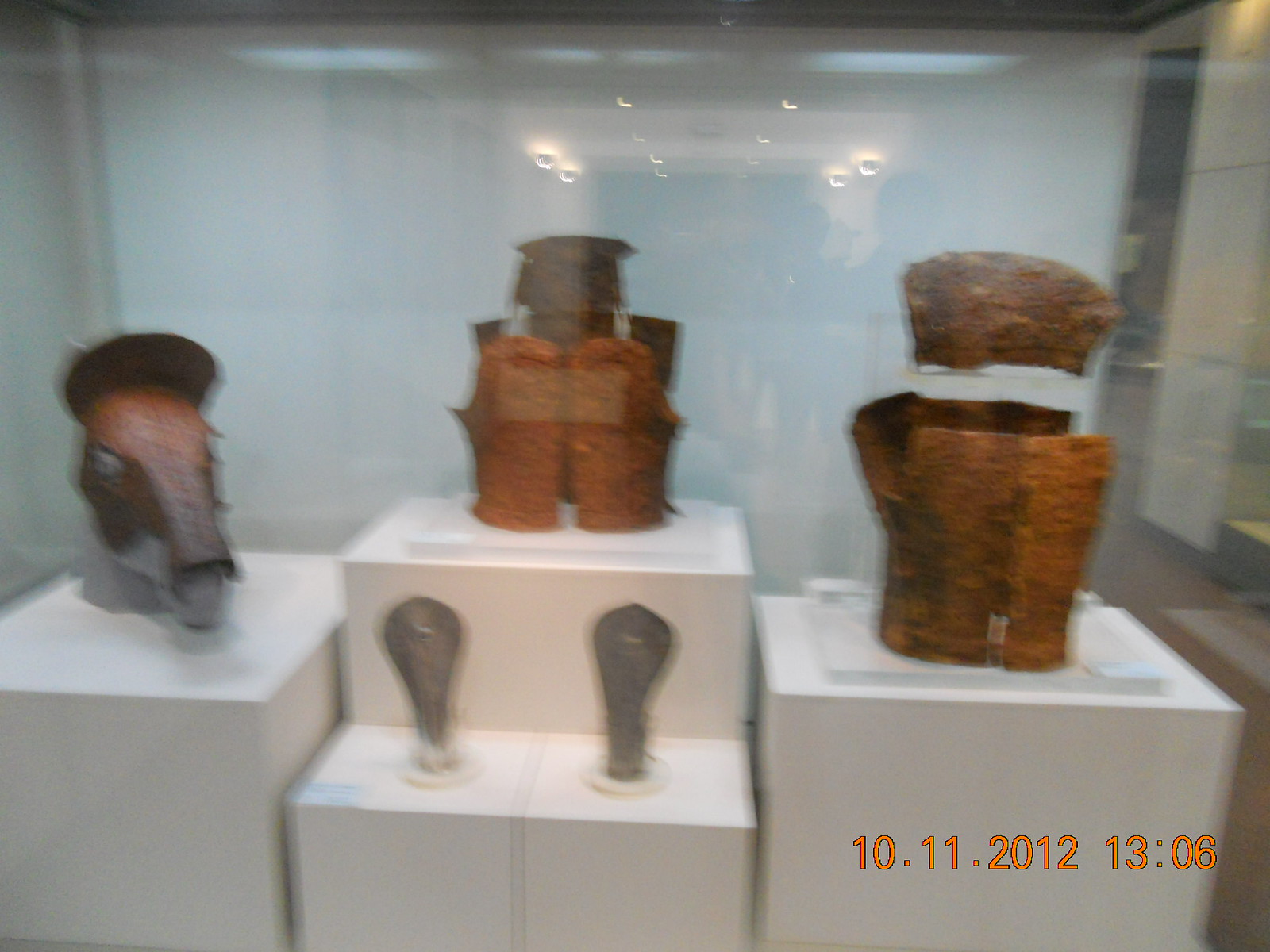This indoor photograph, taken on October 11, 2012 at 13:06, shows a dimly lit museum display case. Encased in glass, the slightly blurry image reveals several artifacts arranged on white boxes of varying heights. Dominating the left side of the display, a horse's head, covered in some form of armor, is visible in profile. Additional objects, possibly including pieces of armor or relics, are positioned centrally and towards the right, though their details are obscured by the blurriness. The artifacts, predominantly brown and gray in color, appear rusted or corroded. The low light conditions and reflections on the glass further obscure the clarity of the photograph. Orange text in the lower right corner of the image displays the timestamp "10.11.2012.13:06."